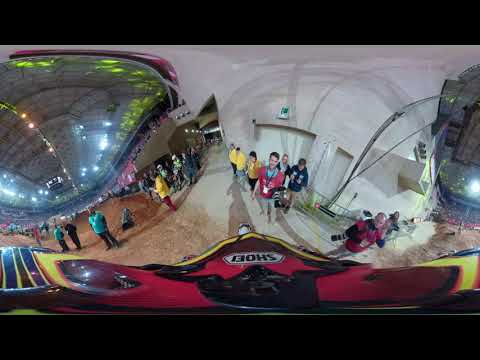The image has an upper and lower black border, framing a central distorted and stretched picture. The scene appears tilted and may have been captured through a specialized lens, possibly a fisheye lens. The primary composition features two bubble-like sub-images on the left and right. 

On the left, a circular area with a dirt floor is visible, suggesting an open or outdoor setting with a roof overhead. People are scattered in both the foreground and background, forming an arc around what seems to be a grandstand filled with seated spectators.

On the right, another section of the image includes doorways in the background and people standing in the foreground, some facing the viewer and others facing different directions. This portion is also distorted, contributing to the overall warped appearance.

The bottom third showcases the stretched front of a vehicle, likely a motorcycle, extending from one edge of the image to the other. It is red and black in the middle, with bulging, yellow ends. The letters "S-H-O-E-I" are imprinted upside down on the vehicle. People in various colored shirts—yellow, red, blue, and black—are gathered around, forming two arcs. Among them, a photographer with a news-style camera can be seen.

Additionally, behind the central group of people, a large doorway with a green exit sign is visible, leading to what seems to be another dome-like structure on the far right. The entire scene appears somewhat disjointed and surreal, suggestive of a reflection or digitally altered image.